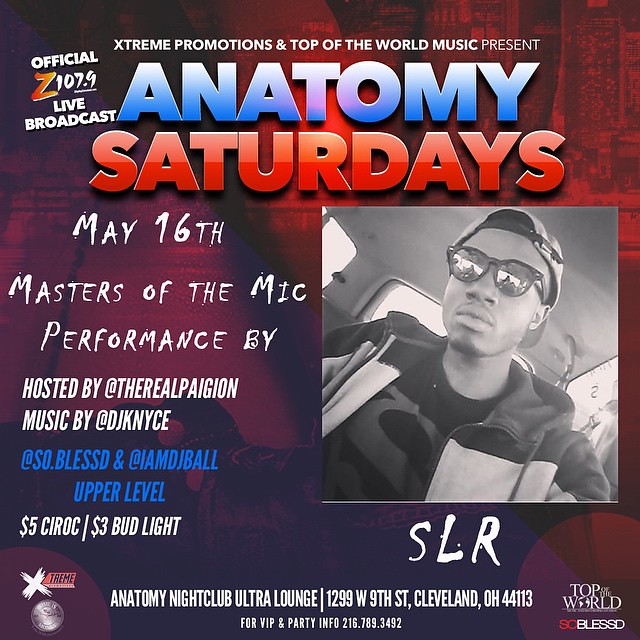This poster, set against a predominantly red background with accents of purple, features blue, red, and white text promoting a live concert. At the top, it reads "Extreme Promotions and Top of the World Music Present Official Z107.9 Live Broadcast." Below this, "Anatomy Saturdays" is highlighted in large blue letters, followed by the date "May 16th" and the event title "Masters at the Mic." The advertisement announces a performance by SLR, hosted by The Real Pajeon, with music by DJ Nice. The event will be held at So Blessed and IMJ Ball on the upper level. Drink specials include $5 Ciroc and $3 Bud Light. A slanted image on the center right features a person wearing sunglasses and a cap. At the bottom, in all white capital letters, are the details: "Anatomy Night Club Ultra Lounge, 1299 West 9th Street, Cleveland, Ohio, 44113." For VIP and party information, the poster provides a contact number: 216-789-3492.